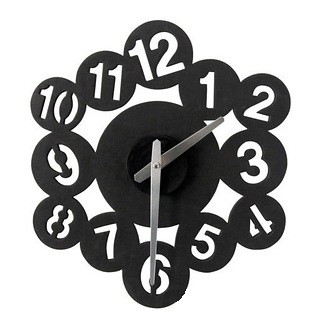This product photo features an abstract, modern clock set against a plain white background. The clock is constructed from thin black metal, giving it a sleek and stylish appearance. At the center is a solid black circle, where the hands of the clock, in stainless steel color, are positioned with the longer hand pointing to six and the shorter hand towards two. Surrounding the central circle are smaller black circles with white numbers, representing the hours. These smaller circles are creatively arranged, not in a perfect circle but in a somewhat jumbled and whimsical fashion. Some circles stick out further, while others are closely nestled, creating a dynamic and funky look. This distinctive design makes it an eye-catching piece of functional art, perfect for modern decor.